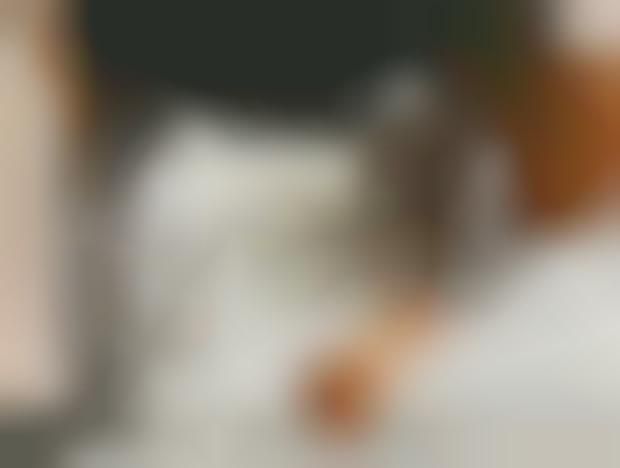The image is a completely blurred horizontal rectangle with indistinguishable features. Dominant colors include a deep blue or brownish blur resembling a tree or hallway on the left side, extending from the top to about 7/8 of the height. At the center-bottom of the image is a white, cloth-like object, and above it, the top center is primarily black, potentially indicating a room or hallway. An orange hue appears as a blob towards the middle, spreading towards the upper right, possibly forming an object or vessel with a white top. There are elements that might suggest the presence of a person holding an object, but this is unclear. Additionally, a white vertical rectangle is noted in the middle center-left, adding to the array of blurred colors and shapes that could be depicting various objects.